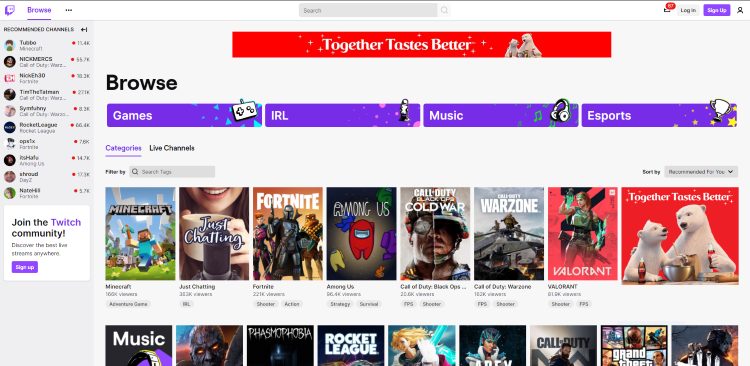The image depicts a screenshot from the streaming platform Twitch, featuring a clean, light-themed interface. Dominating the topmost section of the page, a centrally placed search bar is ready for user input. In the top right-hand corner, two buttons provide quick access to logging in and signing up, respectively.

The header of the webpage showcases four horizontally aligned selection options: "Games," "IRL" (In Real Life), "Music," and "Esports." Below this header, a series of game covers are displayed, including popular titles such as Call of Duty, Minecraft, Rocket League, and Grand Theft Auto.

On the left side of the page, a list of various different channels is visible, each accompanied by their respective names and thumbnail images. In the very top-left corner, the recognizable Twitch icon—a purple chat bubble—sits prominently, next to a purple "Browse" button, encouraging user exploration.